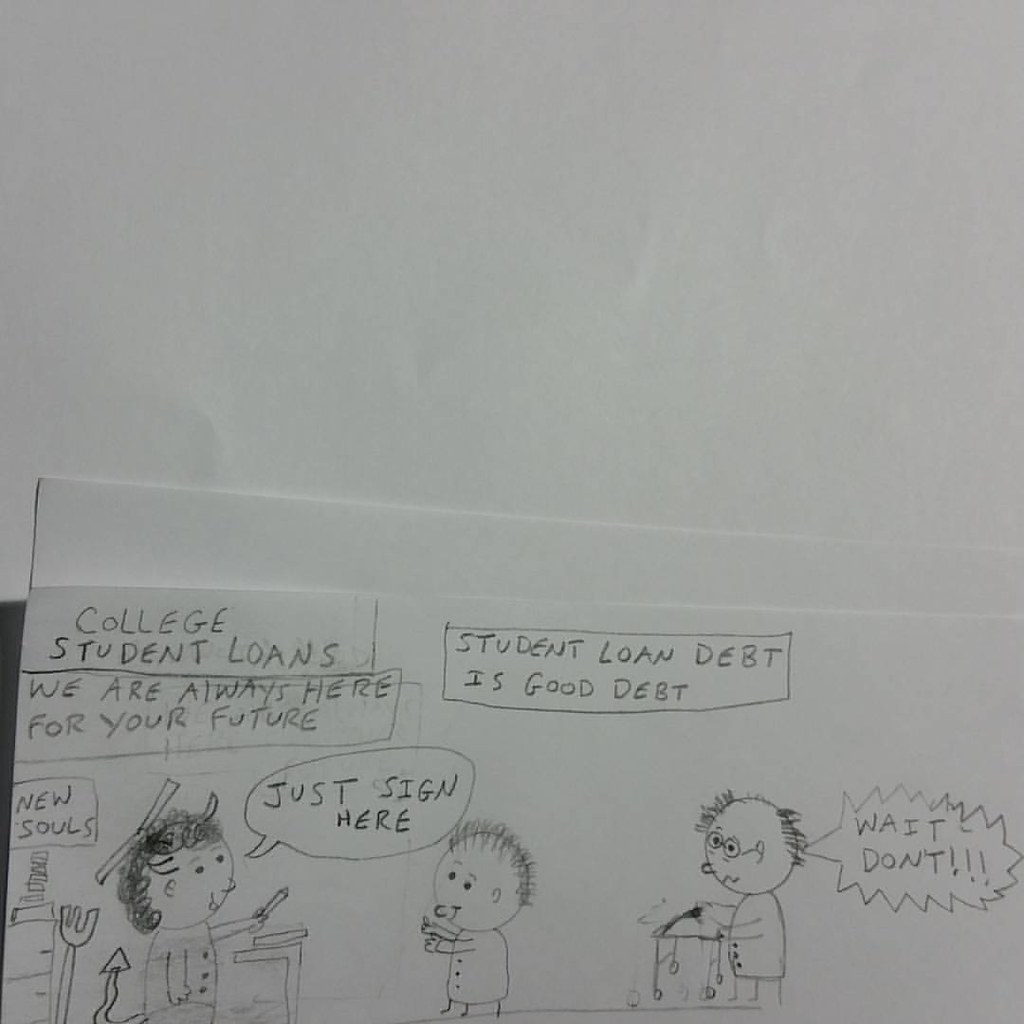This black-and-white comic occupies the bottom third of the image, with the top two-thirds being a blank white space. The comic is a satirical take on college student loans. At the top, it states in black font: "College Student Loans. We are always here for your future. Student loan debt is good debt." The scene features a cartoonish secretary with devil horns, a devil's tail, and a pitchfork, standing behind a sign labeled "New Souls." She extends a pen towards a young boy, urging, "Just sign here." Behind the boy, an older man with a walker, looking frazzled and nervous, exclaims, "Wait, don't!" The overall illustration humorously critiques the predatory nature of student loan practices.